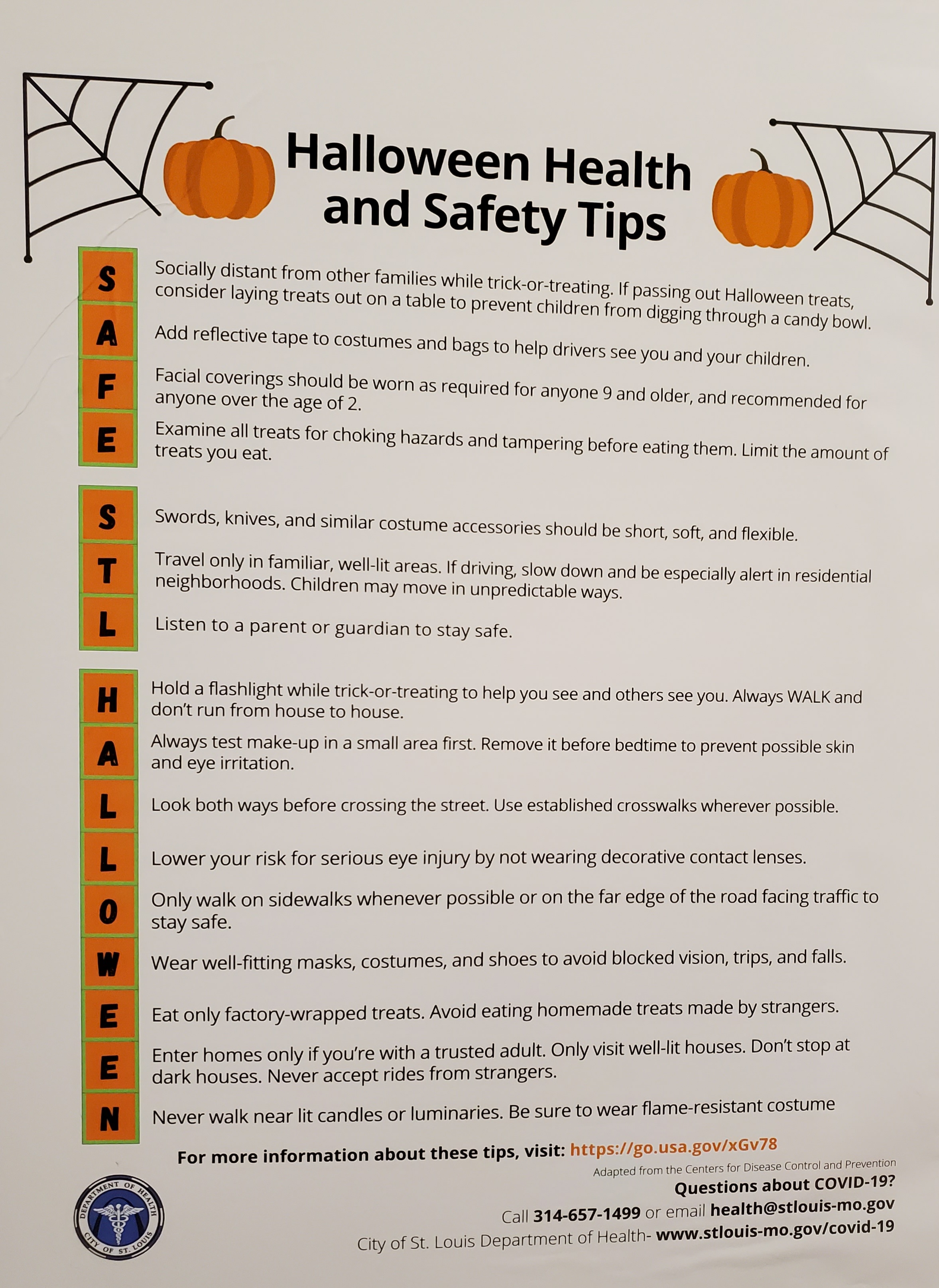This flyer, issued by the Department of Health for the city of St. Louis, features Halloween Health and Safety Tips prominently displayed in bold between two pumpkins on a manila paper background. Spiderweb designs in the top left and right corners add a festive touch to the layout. The flyer uses block letters vertically down the page to spell out SAFE, STL, and HALLOWEEN, each representing a series of safety precautions:

- SAFE: Socially Distant, Add Reflective Tape, Facial Coverings, Examine All Treats.
- STL: Swords and Knives Should Be Short, Soft, and Flexible; Travel Only in Familiar Neighborhoods; Listen to Parent or Guardian.
- HALLOWEEN: A comprehensive acronym with guidelines such as holding a flashlight while trick-or-treating, testing makeup beforehand, and wearing flame-resistant costumes.

The content provides detailed advice for both children and guardians to ensure a safe Halloween, such as staying socially distant, adding reflective tape to costumes, wearing facial coverings, traveling in well-lit areas, and examining treats for safety. Additional safety tips include: always looking both ways before crossing the street, using crosswalks, avoiding decorative contact lenses, only eating factory-wrapped treats, and never accepting rides or entering homes of strangers.

The flyer also includes a section for further information, directing readers to more resources available on the City of St. Louis website. For COVID-19 related questions, it provides contact information including a phone number (314-657-1499) and an email (health@stlouis-mo.gov).

An emblem for the Department of Health is found at the bottom, completing the Halloween-themed safety advisory in orange and black font, reinforcing the urgency and significance of these guidelines.